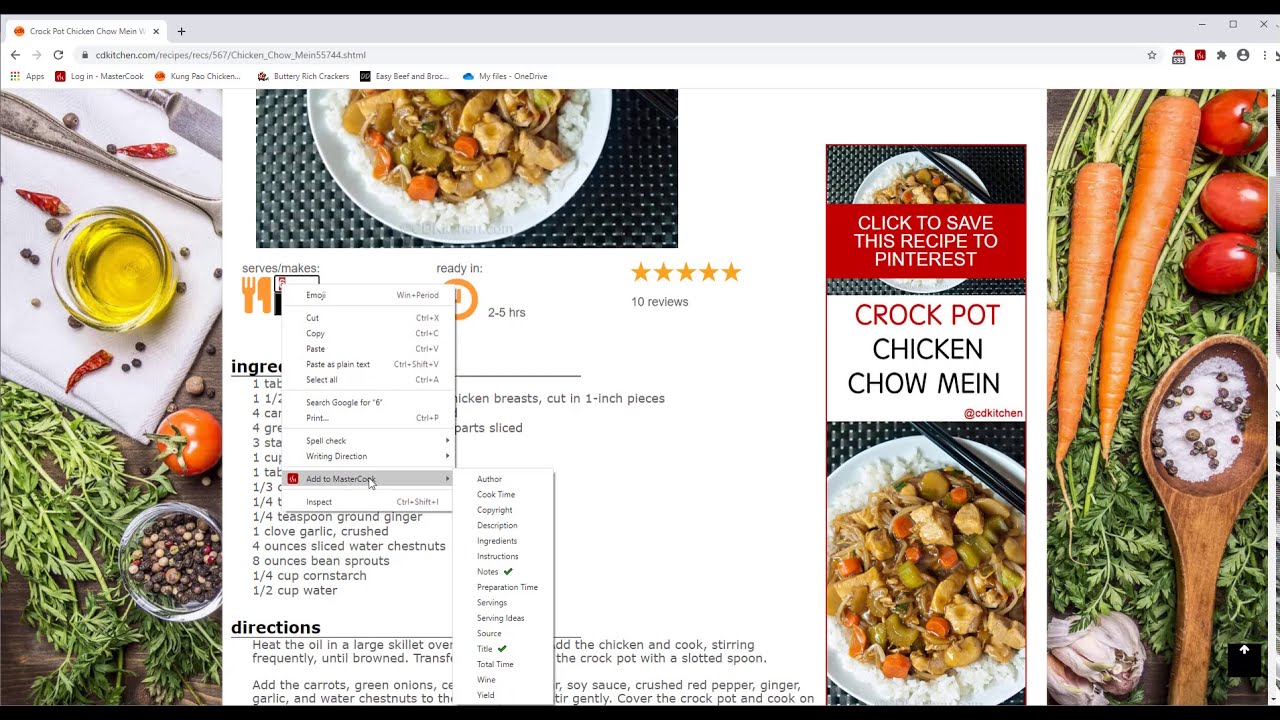**Screenshot Description: Detailed Overview of a Cooking Website**

The screenshot captures a webpage from CDKitchen, specifically showcasing a recipe for Crock-Pot Chicken Chow Mein. The web browser interface includes an "Apps" button on the left-hand side, alongside familiar navigation options such as back, forward, refresh, and login buttons. Other elements visible in the interface are "MasterCook," "Kung Pao Chicken," "Party," "Ritz Crackers," "Easy Beef and Broccoli," and links to "My Files" and "OneDrive."

At the top right corner, the browser interface displays icons for minimizing, maximizing, and closing the window, with an "Adblock Plus" button showing a count of 593 blocked items. There are a few additional, unrecognized icons present in the toolbar as well.

The main web content is centered around a recipe for Crock-Pot Chicken Chow Mein, indicated by the URL which reads "cdkitchen.com/recipes/rex567/chicken_chow_mein5574sthtml." The page features an interactive option where a user has left-clicked to add the recipe to "MasterCook," displaying further prompts to input information such as author, copyright, instructions, notes, preparation time, serving ideas, source title, total time, wine pairings, and other details. This menu partially covers the actual recipe instructions.

Visible parts of the webpage include a section with directions, although it is difficult to read because of the overlaying menus. There is a prompt for saving the recipe to Pinterest, accompanied by two images of Chicken Chow Mein at the top and bottom of the page. An advertisement is also present, and beneath the partially obscured ingredients list, the recipe boasts ten reviews with an average rating of five stars, indicating it is ready in 2 to 5 hours and detailing serving sizes.

Additionally, on the left side of the page, there are images of basil, nuts, tomatoes, olive oil, and peppers, contributing to the culinary theme of the website.

Overall, the screenshot provides a comprehensive yet somewhat obstructed view of the recipe page, complete with web browser toolbar details and additional cooking-related imagery.